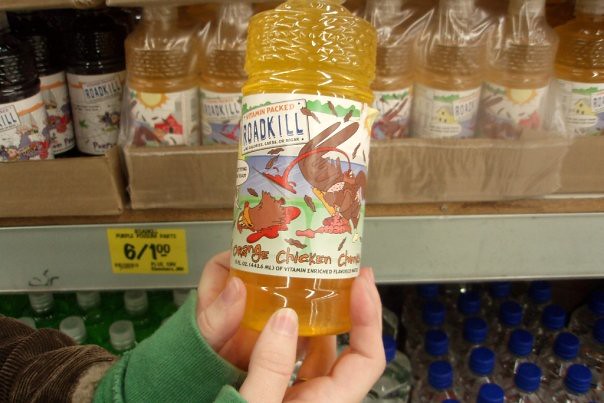A detailed photo shows a person in green sleeves holding a plastic bottle of juice with a yellowish-amber liquid, titled "Vitamin Pact Roadkill Orange Chicken," which is likely the flavor. The bottle has a clear, cartoony label featuring a graphic depiction of a dead chicken with another chicken attacking it, accompanied by blood and a license plate that says "Roadkill." The background of the label includes green grass and blue skies. The scene is set in a store, evident from the surrounding inventory shelves filled with cases of these bottles placed in a large box. The price displayed on the shelf is six bottles for one dollar. The photo highlights both the bottle and the store setting, providing a close-up perspective of the detailed and somewhat graphic label.